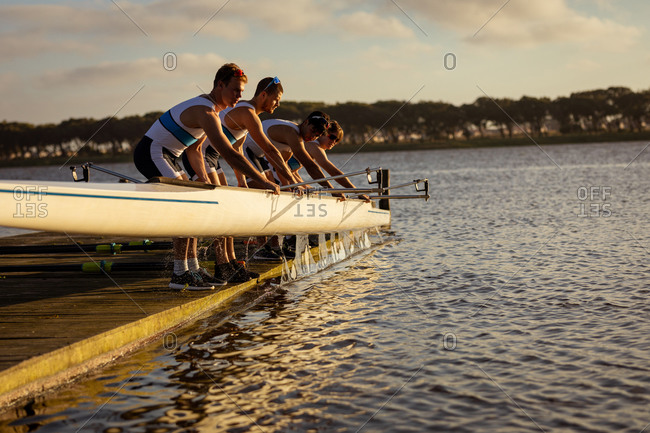The image depicts a serene scene at a river pier, with clear blue skies accented by a few white clouds and a distant tree line. The pier is positioned on the left side, extending out into the water which has a grayish-blue hue with gentle waves. On the pier, four men are engaged in maneuvering a white canoe with a green line on its body. All four are uniformly dressed in white sleeveless jerseys featuring a blue stripe across the chest and black shorts with white stripes down the sides. Their stance is bent over, facing the right, with both hands gripping the canoe—right hand on the outer side and left hand on the inner side. The boat, inscribed with an upside-down "S-E-T," appears to be either being pulled out of the water or put back in. Metal brackets are attached to the pier, aiding in their task. The men are also wearing tennis shoes and are uniformly positioned, depicting a coordinated effort in handling the canoe.